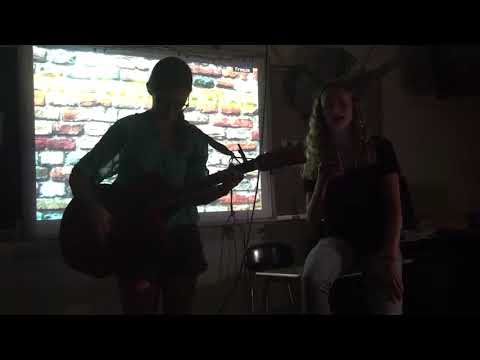The image depicts a dimly lit performance scene inside what appears to be a classroom. At the center of the scene is a large projector screen displaying a multicolored brick wall composed of red and yellow bricks. In front of this screen are two young Caucasian women engaged in a musical performance. On the left, a woman with glasses and tied-back brown hair dons a mint green shirt and black shorts. She is in the midst of playing an acoustic guitar, her focus directed downward towards the instrument. On the right, a woman with long, wavy blonde hair, clad in light white pants and a short-sleeved black shirt, is perched on a student desk with an attached chair. She sits half-on, half-off the desk, one arm raised, her mouth open in song, and her eyes closed. Classroom desks and chairs are faintly visible in the dark surroundings, adding to the intimate setting of the performance.